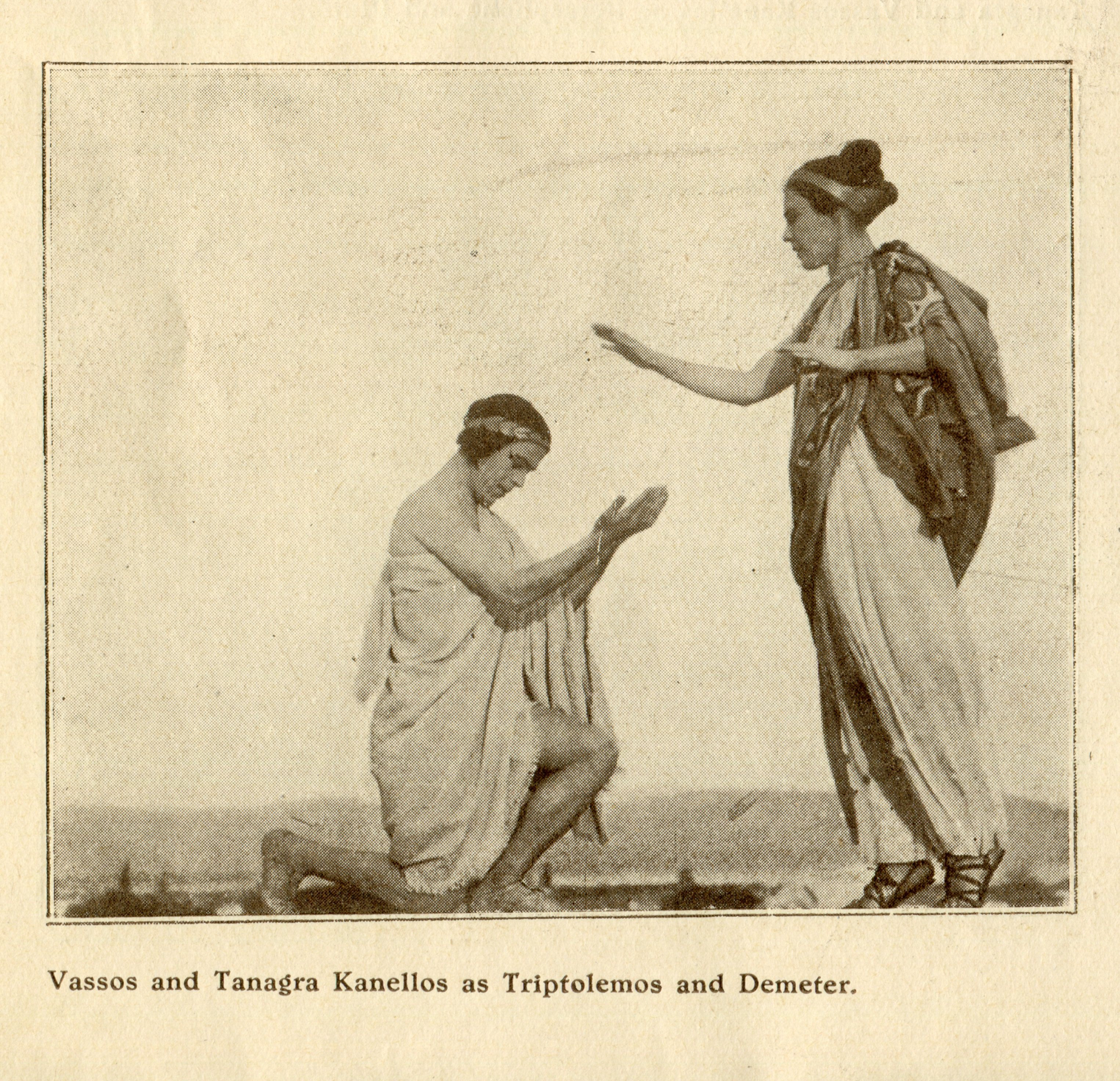This image is a weathered, yellowed photograph, with a black outline forming a square on a light peach or pink background. Within the square, a man and a woman are depicted in classical attire. The man, positioned on the left, is kneeling on one knee with his palms upraised toward the woman. He wears a white toga and a metal or gold wreath in his hair. His gaze is directed downward. The woman stands to his right, her hair styled in a bun, and she dons a colorful shawl over her shoulders with white, billowing pants and sandals. She gazes down at the man, her right hand extended with the palm down, almost blessing him. Her left hand is positioned slightly in front of her. In the distance, faint hills can be seen. The bottom of the image features black text on a larger, pink border, reading "Vassos and Tanagra Kanellos as Tryptolomas and Demeter."